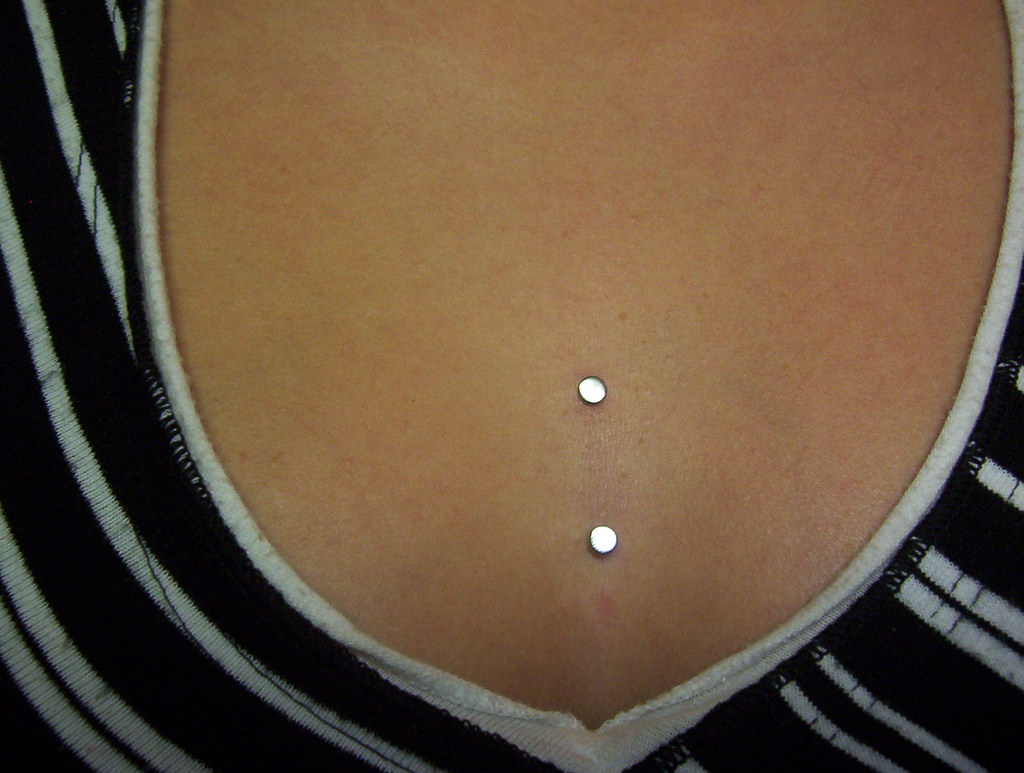The image is a close-up of a woman's chest, focusing on a unique sternum piercing arrangement with two metallic silver studs. The skin is fair with a slight tan, and you can notice some mottled red areas. The woman is wearing a black knit top, characterized by horizontal white stripes, which has a low scoop or V-shaped neckline that cuts right above the breast level. The two round silver discs, resembling small watch batteries, are spaced about an inch or two apart and appear embedded directly on the breastbone, centrally located in the image. This simple, detailed composition effectively highlights the distinctive piercings against the striped pattern of the shirt and the natural skin tone.